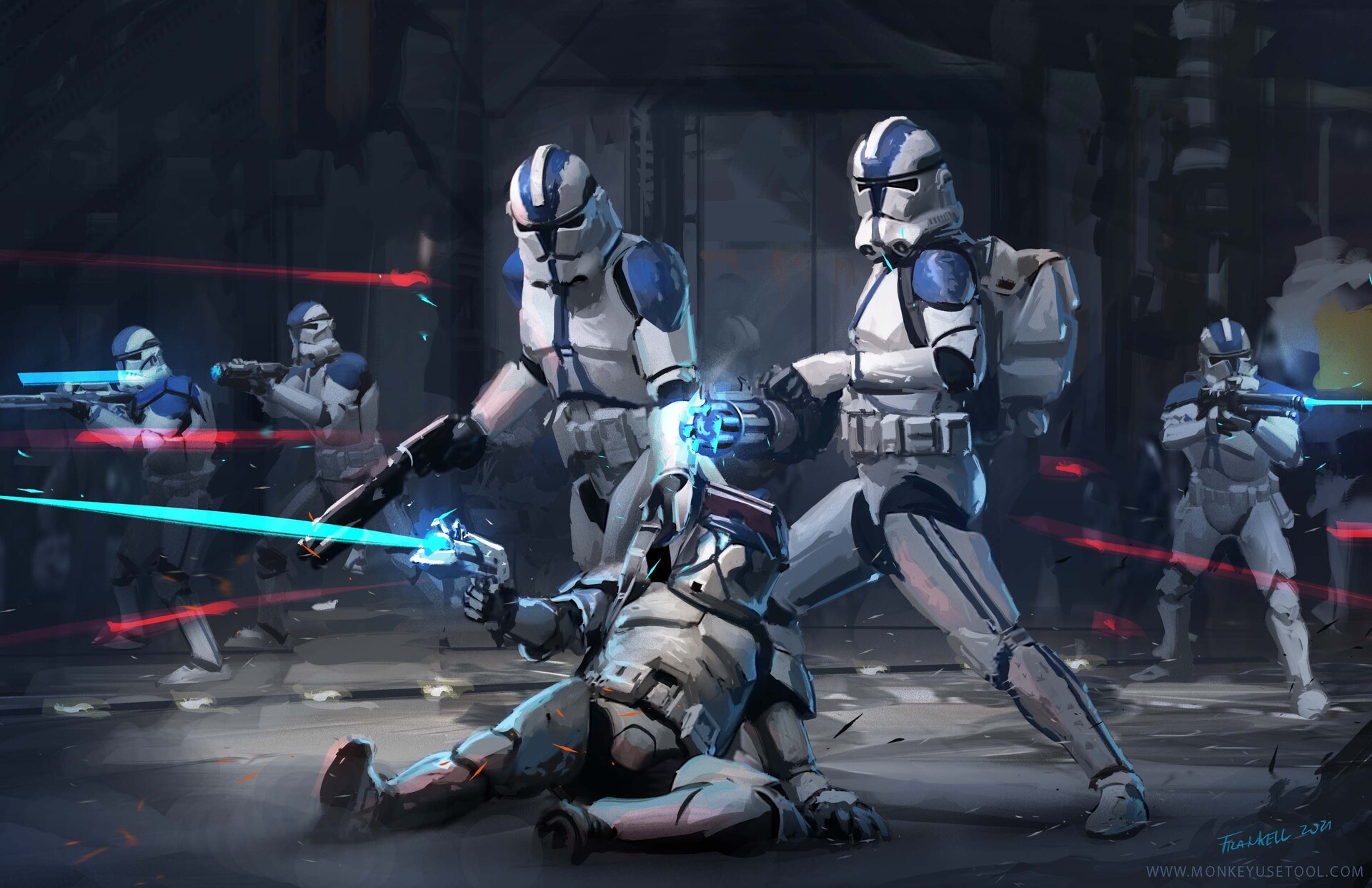The image is an intricate piece of artwork depicting a dramatic scene from Star Wars. Signed illegibly in teal paint at the lower right corner, the painting features a dark, futuristic interior with a metallic wall embedded with complex machinery and scattered debris. Central to the scene are multiple Imperial Stormtroopers, adorned in white plate armor with distinctive blue stripes running up the center of their masks, chest pieces, and shoulder pads.

In the foreground, two Stormtroopers are focused on a fallen comrade. One of them, equipped with a long black blaster, appears to be assisting the downed trooper. This downed Stormtrooper is partially upright, defiantly firing a neon blue energy beam from his weapon. To the right, another Stormtrooper wields a turret-like, spiraling machine gun, emitting intense blue light beams.

In the background, three additional Stormtroopers are engaged in combat. They are positioned against the metallic wall, firing their energy weapons that shoot blue and red rays in various directions, adding to the chaos and intensity of the scene. The overall ambiance of the artwork is dark, invoking a sense of tension and urgency as these armored figures navigate through what appears to be a ravaged futuristic battleground.